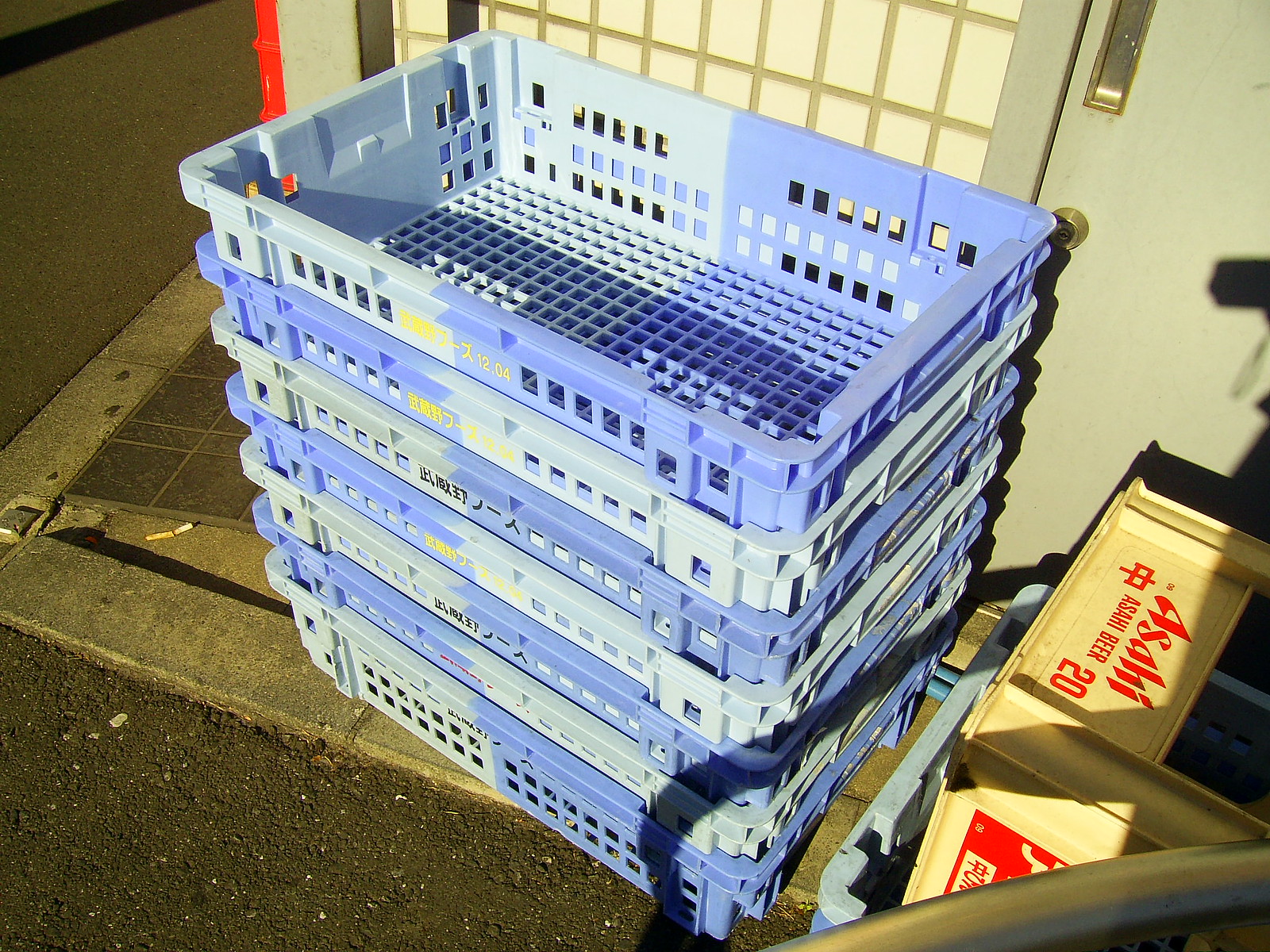In this bright, outdoor close-up photograph, we see a scene featuring a portion of a gray building with a shop door adorned with white and gray squares. In front of the door, there are seven to eight light blue plastic crates stacked high, each perforated with square holes. Some of the crates have Japanese kanji writings in black and yellow on their sides. To the right of this tall stack, there is another smaller pile of similar crates, alongside a single white crate containing miscellaneous items. The ground is a mix of black asphalt and poorly laid tiles or pavers, dotted with gravel and dirt. Notably, a lone cigarette butt is discarded on the pavement near the stacks. A metal bar protrudes from the lower right corner of the image, and the building structure includes a slight hint of red on one corner.